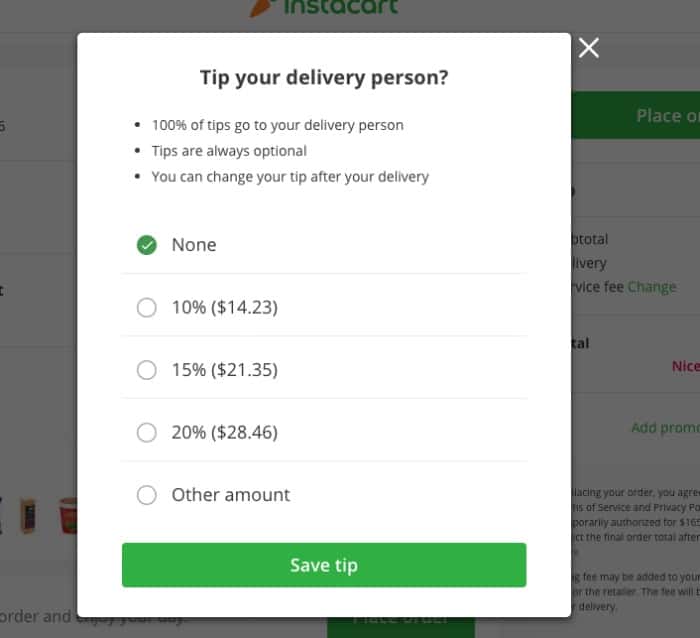This image is a screenshot of a webpage displaying a prominent pop-up window on the Instacart platform. In the background, a partially visible, darkened webpage shows a predominantly white interface with a green button at the top left, accompanied by some descriptive text. The top of the page features the Instacart logo—a green wordmark "Instacart" with an orange, cartoon-style carrot.

The pop-up window is centered and takes up most of the frame, with a white background casting a slight dark grey shadow behind it. At the top of the pop-up, black text reads, "Tip Your Delivery Person," followed by three bullet points explaining:

1. "100% of tips go to your delivery person."
2. "Tips are always optional."
3. "You can change your tip after your delivery."

An 'X' icon, representing the option to close the pop-up, hovers above and to the right of the rectangle.

Below the bullet points, five separate tipping options are presented, each divided by thin grey lines. The first option, labeled "None," is selected, indicated by a green circle with a white checkmark. The subsequent options display grey circles and are labeled as follows:

- "10% ($14.23)"
- "15% ($21.35)"
- "20% ($28.46)"
- "Other amount"

At the bottom of the pop-up, a green button with slightly rounded corners spans almost the entire width of the window. The button features white text that reads "Save Tip," with a capital "S" in "Save" and a lowercase "t" in "tip."